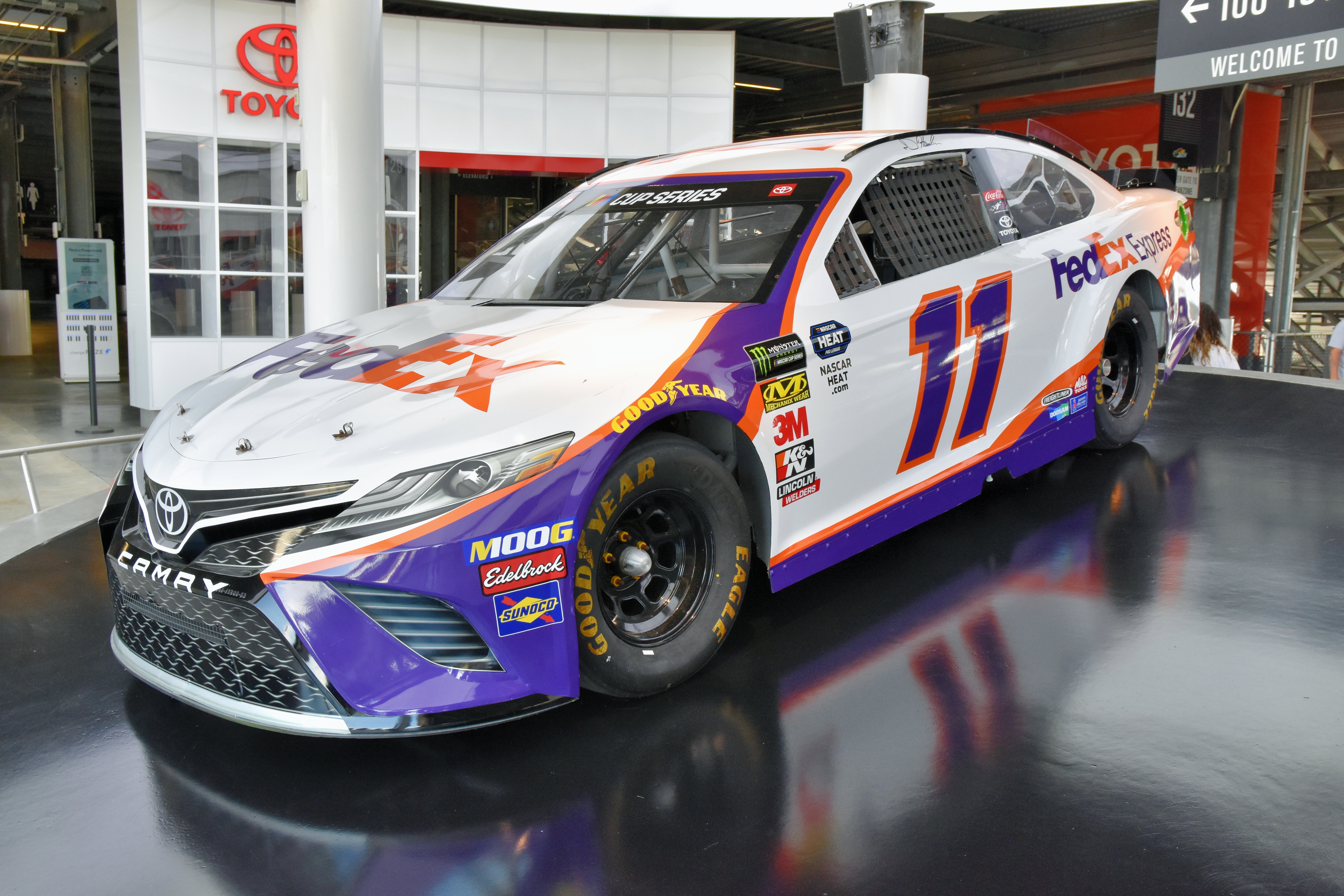This image is a professionally taken, brightly lit photograph of a Toyota-sponsored stock car being showcased indoors at a Toyota facility. The background prominently features a red Toyota sign on a white wall, alongside a gray sign with white letters that reads "Welcome To." The race car itself is primarily white, accented with purple and orange trim, and prominently displays the number 11. The car features numerous sponsor logos, including FedEx, FedEx Express, Explosives, 3M, Sunoco, Monster Energy Drink, and Moog, indicating a strong sponsorship presence. The clean and detailed shot suggests that the car is not a pedestrian vehicle but a professional racing car likely used for advertising and promotional purposes. Two distinct white pillars in the background further frame the display scene, contributing to the overall professional presentation.